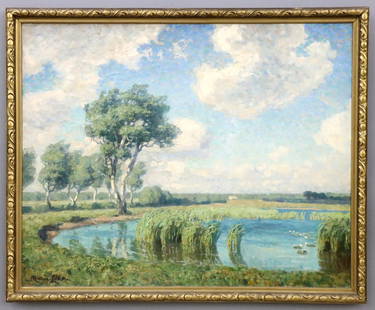This horizontal rectangular image features a detailed and ornate golden frame with carved decorations. Inside the frame is a serene painting of a natural landscape. The upper half of the painting showcases a vast blue sky filled with fluffy white and hints of gray clouds. Dominating the lower portion is a blue lake bordered by lush green grass and bushes, with some lily pads visible on the water's surface. On the left side of the painting, a cluster of trees stands out, including one particularly tall tree that reaches towards the sky. The lake reflects portions of the sky and nearby trees, adding to the tranquil atmosphere. The background surrounding the frame is solid gray, emphasizing the artwork's vibrant colors and intricate details.